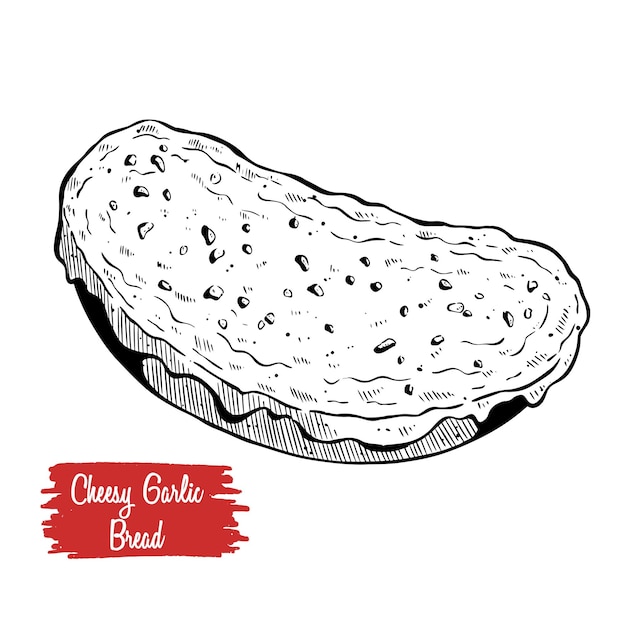This is a detailed black and white line drawing of cheesy garlic bread set against a white background. In the bottom left corner, there's a bright red rectangular streak with fringed edges on the sides and flat top and bottom, with the text "cheesy garlic bread" elegantly written in cursive white lettering. Above this text, the illustration depicts an oval or half-moon shaped piece of bread. The bread has a textured crust illustrated through streaks of lines, and melty cheese oozing over the sides. Speckles and chunks, presumably bits of garlic, are nestled in the cheese, giving a detailed and appetizing portrayal of cheesy garlic bread.